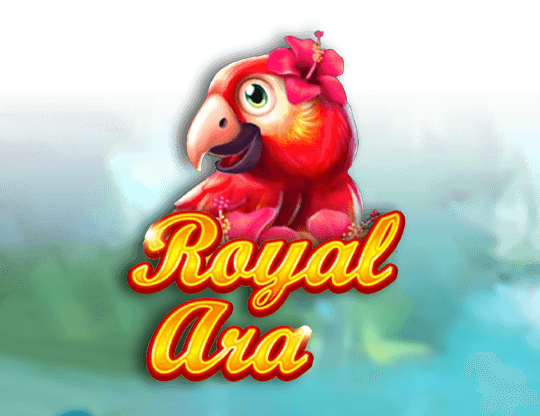The image showcases a detailed, cartoon illustration of a smiling red parrot with green eyes and yellow-blushed cheeks. The parrot is facing left, adorned with a pink or magenta hibiscus flower where a person's ear would be. The beak is a distinct light red with a dark mouth underneath, slightly open to reveal a red tongue. The background of the image is a mix of green tones, hinting at a tropical forest, fading to white at the top, giving a blurry and out-of-focus appearance. Below the parrot, in a large, cursive script, metallic gold font with a red outline, it reads "Royal Ara." The overall effect is vibrant, with the parrot's varied shades of red and pink standing out against the lush, ambiguous background.